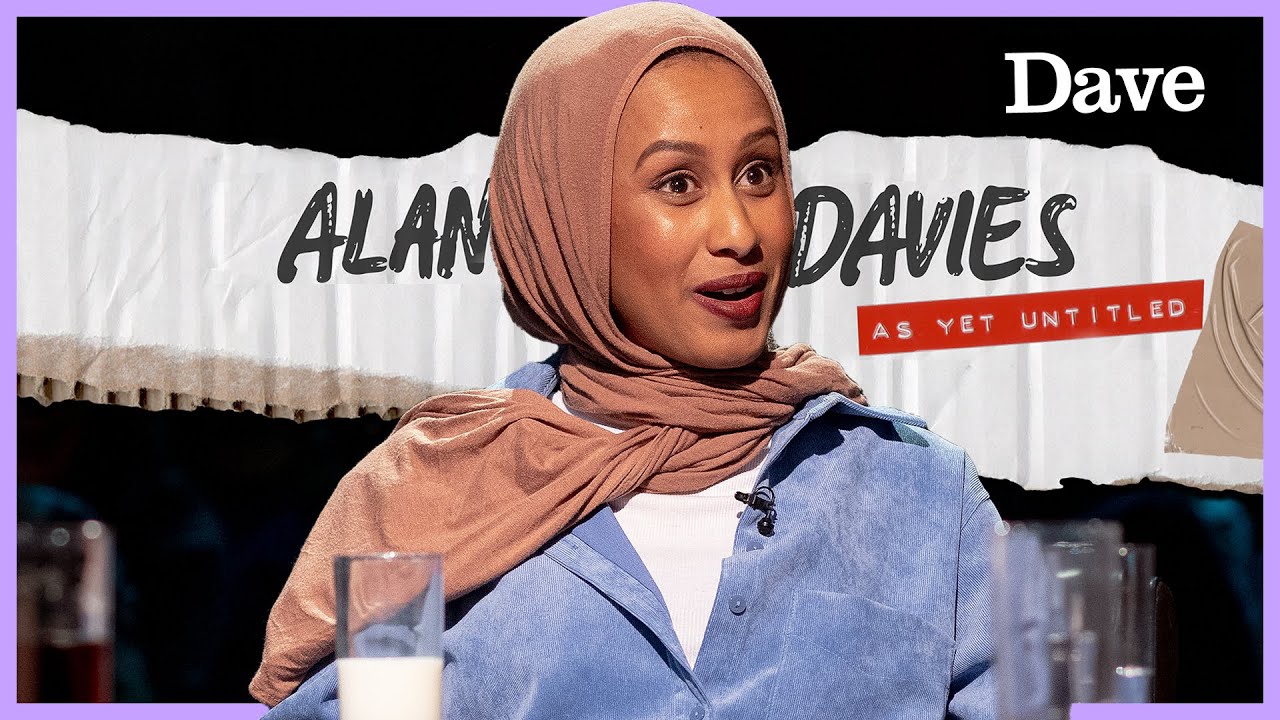In this captivating image, a woman is seated at a table, suggested by the presence of assorted glassware in front of her, including a half-full glass of milk positioned to her right. She faces the camera, with her head turned slightly to her right, revealing a contemplative expression. Adorning her head is a brown scarf that elegantly wraps around her neck, drapes over her right shoulder, and extends across her left shoulder. Her striking appearance is accentuated by her vibrant red lipstick. She is impeccably dressed in a blue long-sleeved button-down shirt layered over a white t-shirt. The backdrop adds intriguing context: in the upper right corner, the word "Dave" is displayed in white font, and a torn piece of cardboard-like material adds texture and depth to the scene.